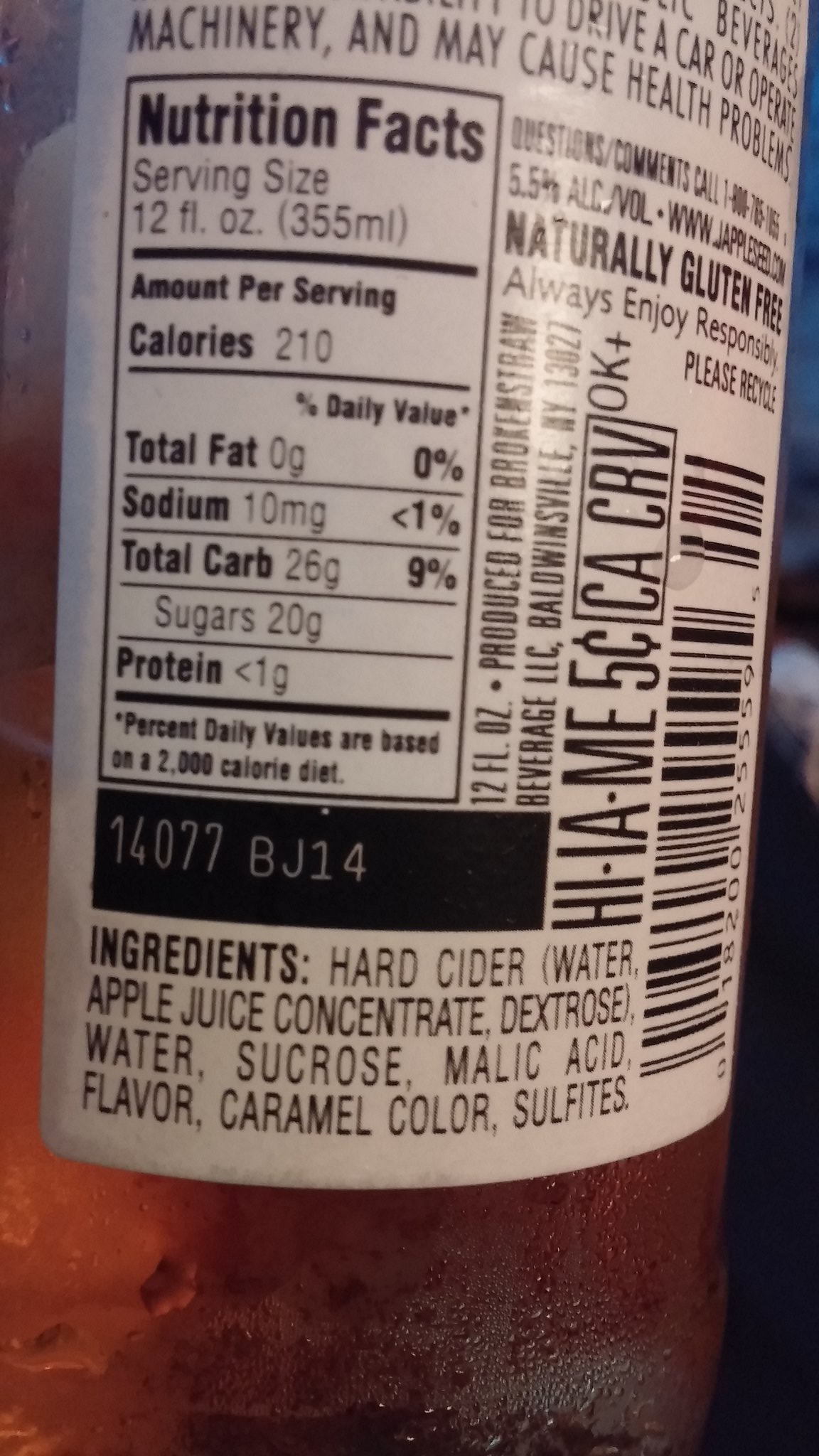This vertically-oriented rectangular image showcases a label on a clear bottle containing a dark liquid. The label prominently displays "Nutritional Facts" at the top, stating that the bottle has a volume of 12 ounces and contains 210 calories. Below, the "Ingredients" section lists the contents as Hard Cider, with further detail provided in parentheses: Water, Apple Juice Concentrate, Water, Sucrose, Malic Acid, Flavor, Caramel Color, and Sulfites. The label also mentions that the product is "Naturally Gluten-Free." Additional text advises consumers to "Always enjoy responsibly" and to "Please recycle." Partially visible text warns against certain activities, indicating it is dangerous to "Drive a car or operate machinery" after consumption, and notes that drinking may "cause health problems."